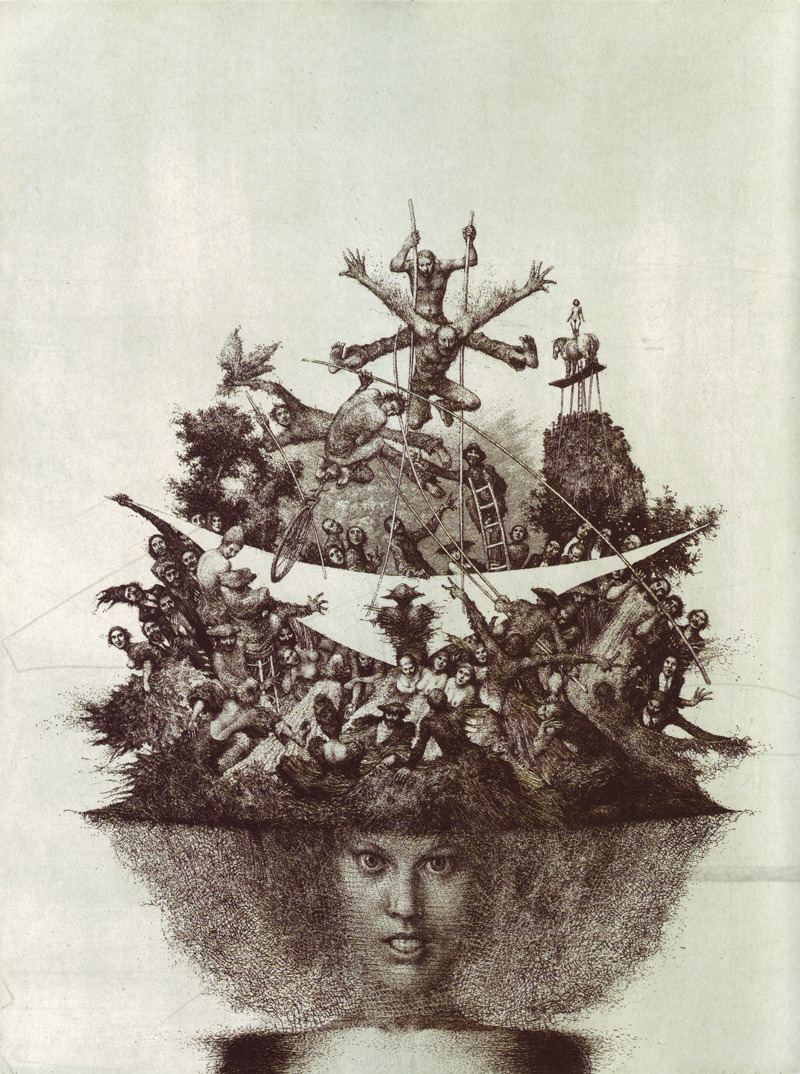This image is a detailed black and white pencil sketch that depicts a woman from her collarbones up to just above her eyebrows, wearing a determined expression with clenched teeth and almond-shaped eyes. Her hair is depicted as enormous and frazzled, expanding out past her shoulders and transforming into a fantastical scene above her forehead. This scene is reminiscent of a lively circus or carnival, featuring a variety of dynamic characters and activities.

Atop her voluminous hair, rows of human figures engage in various acts. On the right, a horse stands precariously on a tall scaffold with a naked lady riding it. A clown climbs a ladder, while acrobats perform daring stunts, including a person on stilts with another figure jumping between their legs. There are individuals lying down, some holding fishing poles or long sticks comparable to those used in pole vaulting, and a unicyclist balancing towards the top. Intriguingly, it almost looks like Jesus is present, holding long sticks, near a tree on the right. 

In the center, a triangular parachute seems poised to catch a falling person. The woman's hair, styled as a wide afro, serves as a nesting area for these surreal and whimsical elements, creating an overall impression of bustling, chaotic energy. The astonishing array of activities provides a window into a vivid, imaginative world, all contained within the confines of this intricate sketch.